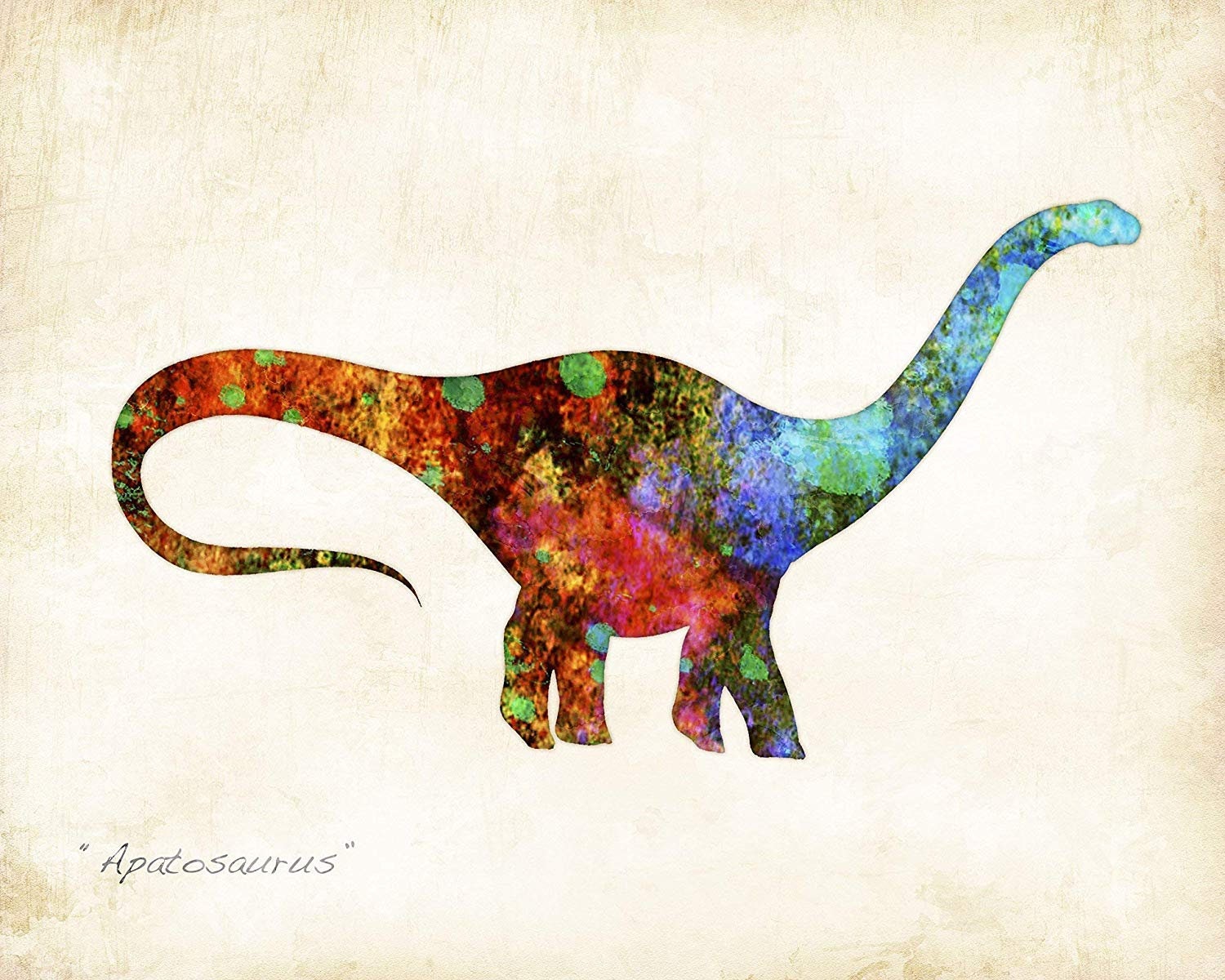This detailed illustration, displayed on what resembles aged parchment paper, features a vibrant portrayal of an Apatosaurus, as indicated by the caption "Apatosaurus" in quotation marks at the bottom left corner. The dinosaur is depicted in a dynamic profile, walking with an extended neck reaching upward to the right and a tail that extends to the left before curling back near its legs in a distinctive J-hook shape. While the outline of the Apatosaurus is precise and likely realistic, the interior coloring is highly artistic, resembling a tie-dye effect with a myriad of colors. The head and neck transition from blue and green to deeper hues, while the body is primarily adorned with orange, red, and green shades. The tail darkens to an almost black color speckled with red, yellow, and green accents. The entire figure is a striking collage of various colors, applied in a manner that emphasizes a lack of uniform patterns, creating a whimsical and captivating visual experience.